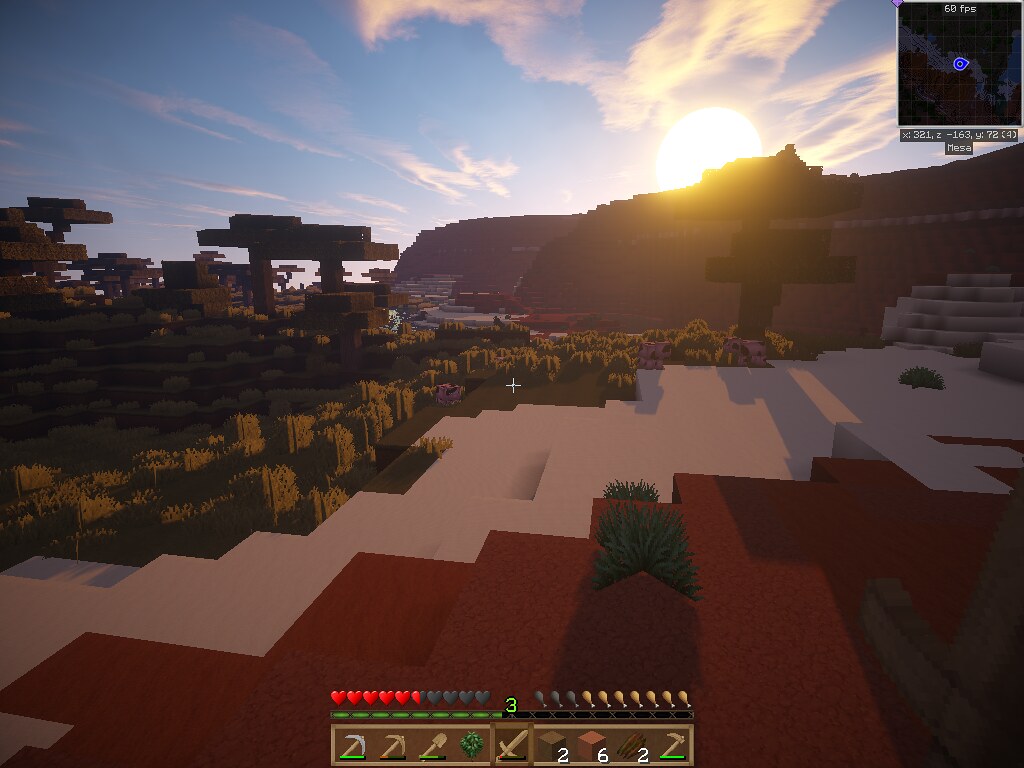This screenshot from a Minecraft game captures a serene daytime scene, evident by the bright blue sky adorned with faint, white clouds and a visible sun. In the top right corner, the screen displays "60 FPS" along with a mini-map. The player's inventory, located at the center bottom, includes a variety of tools and items: a steel pickaxe, a wooden pickaxe, a wooden shovel, a green plant, a wooden sword, two dirt blocks, miscellaneous other blocks, and a sickle. The player's health is at half capacity, while the food bar is approximately three-fourths full. The landscape features a snowy environment with numerous trees, shrubs, and weeds scattered around. Dominating the center of the image are three cows, adding life to this tranquil, wintery scene.